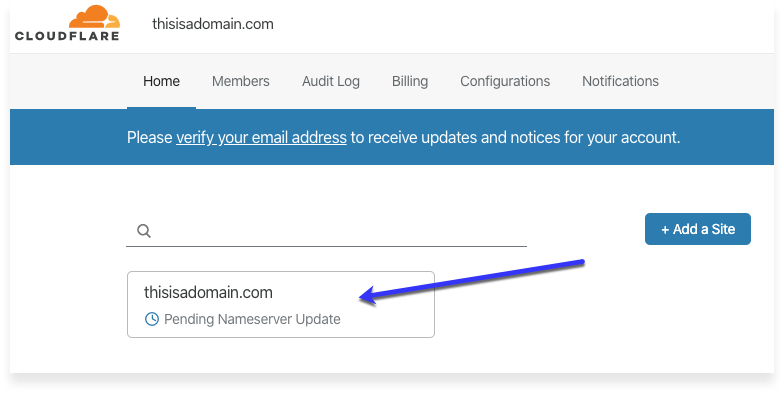The web page features a Cloudflare icon at the top left corner. The icon is predominantly black and features an orange cloud with what appears to be a plane or a starburst within the cloud. Next to the icon, the text reads "this is a domain.com."

The next section of the page is a light gray bar containing six categories in black text: Home, Members, Audit Log, Billing, Configurations, and Notifications.

Beneath this, there's a blue bar with white text that prompts users to verify their email address in order to receive updates and notices for their account.

The main body of the webpage is white. It includes a long search bar where users can enter their email addresses. Below the search bar, there is a rectangular section labeled "this is a domain.com" accompanied by a note indicating a "pending name server update." An arrow from a blue bar labeled "Add a Site" points to this notification, and the background remains white throughout this section.